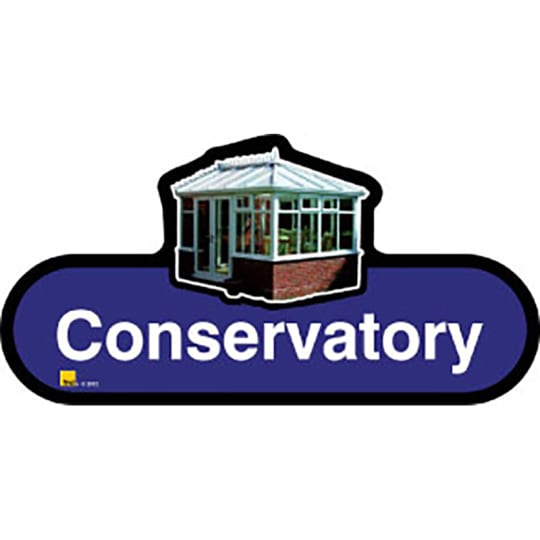The image depicts a detailed logo for a conservatory. At the bottom, there is an elliptical dark blue shape outlined in black, with bold white letters that read "Conservatory." On the lower left corner of this shape, there is a small yellow square, possibly a trademark symbol, with tiny, unreadable letters. Above the text is a stylized depiction of the conservatory itself, featuring a red brick base and a structure made primarily of white-framed glass windows. The building has a white roof, which contrasts with the glass-heavy design, suggesting it may not be a traditional greenhouse. The conservatory includes two large, white-framed, glass double doors; through the windows, chairs are visible inside. This logo likely appears on various advertising materials for the conservatory.